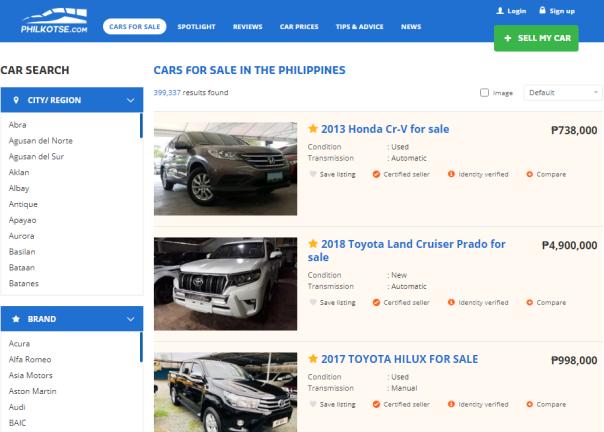The image depicts the website homepage of philcoetzee.com, a platform dedicated to automobile sales and information. At the top of the page, a striking blue banner garners immediate attention. The site offers various sections, including "Cars for Sale," "Spotlight Reviews," "Car Prices," "Tips and Advice," and "News." The "Cars for Sale" section is currently highlighted.

A green pop-up window, marked with a plus sign, appears with the option "Sell My Car." Below this, users can initiate a car search by specifying their city or region and selecting a car brand from a dropdown menu featuring options such as Acura and Audi. 

Centrally displayed, a bold blue header announces "Cars for Sale in the Philippines." Beneath this heading, three cars are listed: a 2013 Honda, a 2018 Toyota Land Cruiser, and a 2017 Honda Hilux. Each vehicle is presented in an individual box with a pinkish background. Accompanying each listing is an actual photograph of the car, situated next to the vehicle's title and a brief description.